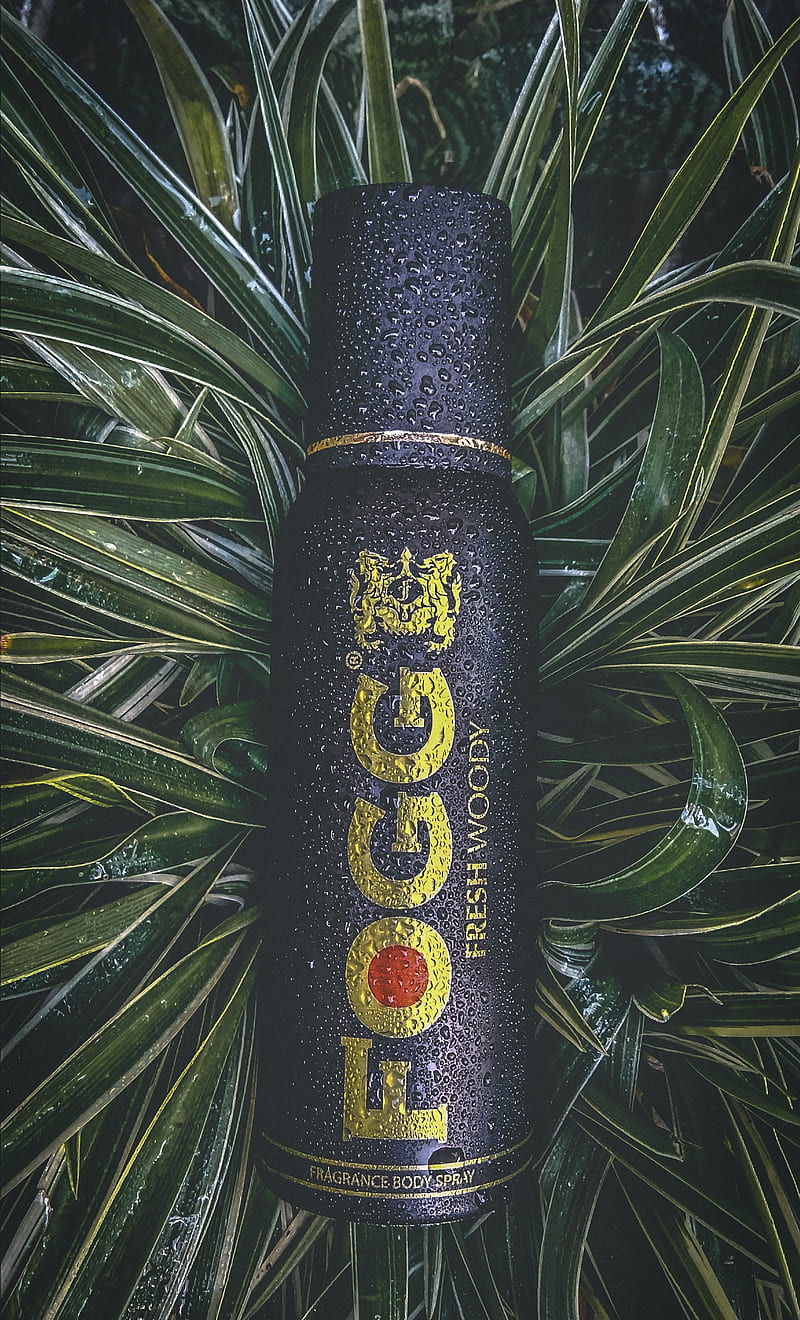The image features a black spray can adorned with gold text, prominently displaying the word "FOGG" in a vertical arrangement. The letter 'O' in "FOGG" contains a solid red circle. Adjacent to the text, there is a gold emblem resembling a medieval crest with two dragons on either side. Below this text, the phrase "Fresh Woody" appears in coordinated gold paint. The can, identified at the bottom as a "Fragrance Body Spray," is capped with a black lid detailed with a thin gold line. The entire surface of the can is wet, covered in droplets of water, and it rests atop a vivid, verdant bed of wet leaves, with the long, thin, dark green foliage streaked with hues of black and yellow.